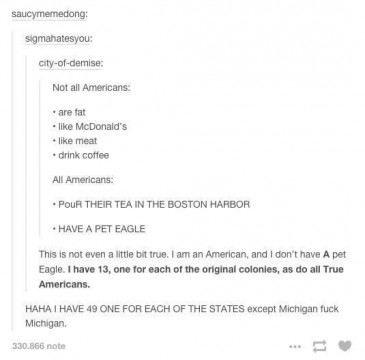The image is a vertically rectangular meme on a white background, featuring a series of satirical statements presented in a structured list. 

At the top left corner, in lowercase black font, the words "saucy memedong:" are written, which is followed by the heading "Sigma hates you:". Below this, the structured list begins:

1. "city-of-demise:"
2. "not all Americans:"
   - The first bullet point states: "are fat."
   - The second bullet point: "like McDonald's."
   - The third bullet point: "like meat."
   - The fourth bullet point: "drink coffee."

Following this, there is another subheading "all Americans:" with its own bullet points:
- The first bullet point, in all capital letters, says: "POUR THEIR TEA IN THE BOSTON HARBOR."
- The second bullet point says: "have a pet eagle."

Underneath these, the text shifts slightly to the left, with more indented statements:
- "This is not even a little bit true. I am an American and I don't have a pet eagle. I have 13, one for each of the original colonies, as do all true Americans." The phrase starting from "I have 13" is in bold black font.
- Following this, in regular black font, it reads: "I have 49, one for each of the states except Michigan." This line ends with an explicit derogatory statement about Michigan.

The overall tone of the meme is satirical, poking fun at stereotypes and exaggerating American cultural tropes.